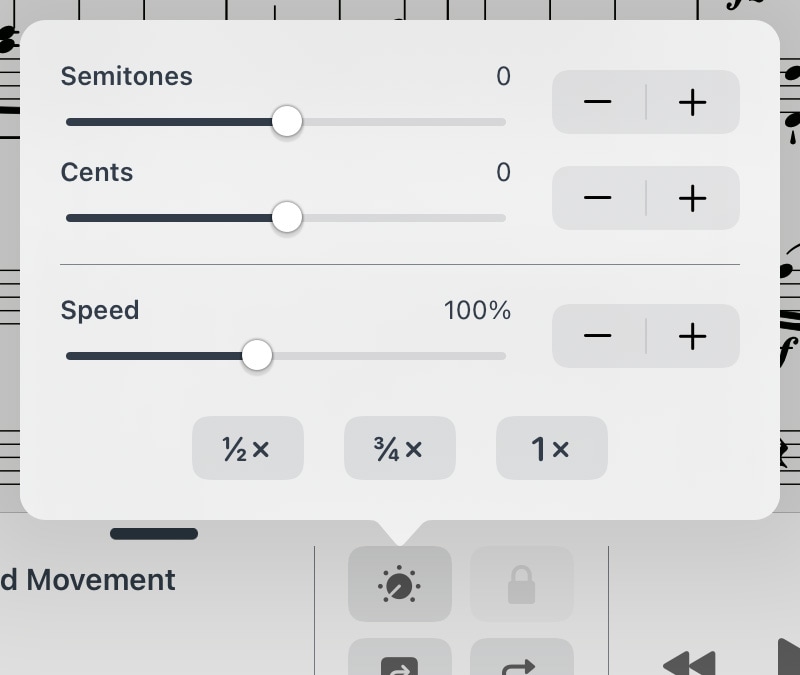The image depicts a pop-up window overlaying a screen, obscuring most of the underlying content. The underlying screen is predominantly gray and black, while the pop-up window is a light gray. The pop-up contains three central elements: 

1. **Semitones**: Accompanied by a horizontal slider bar set at the middle position, indicated by a "0". Adjacent to the slider bar on the right are plus (+) and minus (-) buttons.
 
2. **Cents**: Similarly, this section has a horizontal slider set at the middle, denoted by a "0", also flanked by plus (+) and minus (-) buttons on the right.

3. **Speed**: This section features a horizontal slider positioned in the middle, marked at "100%". It too has plus (+) and minus (-) buttons situated to the right of the slider.

At the bottom of the pop-up are three buttons labeled as follows:

- "0.5×" (indicating half speed)
- "0.75×" (indicating three-fourths speed)
- "1×" (indicating standard speed)

The color palette of the pop-up consists predominantly of various shades of gray, from light to medium gray, with black font providing contrast. The specific function of the pop-up remains unclear, as it does not provide any context, leaving terms like "semitones," "cents," and "speed" somewhat ambiguous in their application. It is also unclear which device (phone, tablet, or computer) or website is hosting this pop-up.